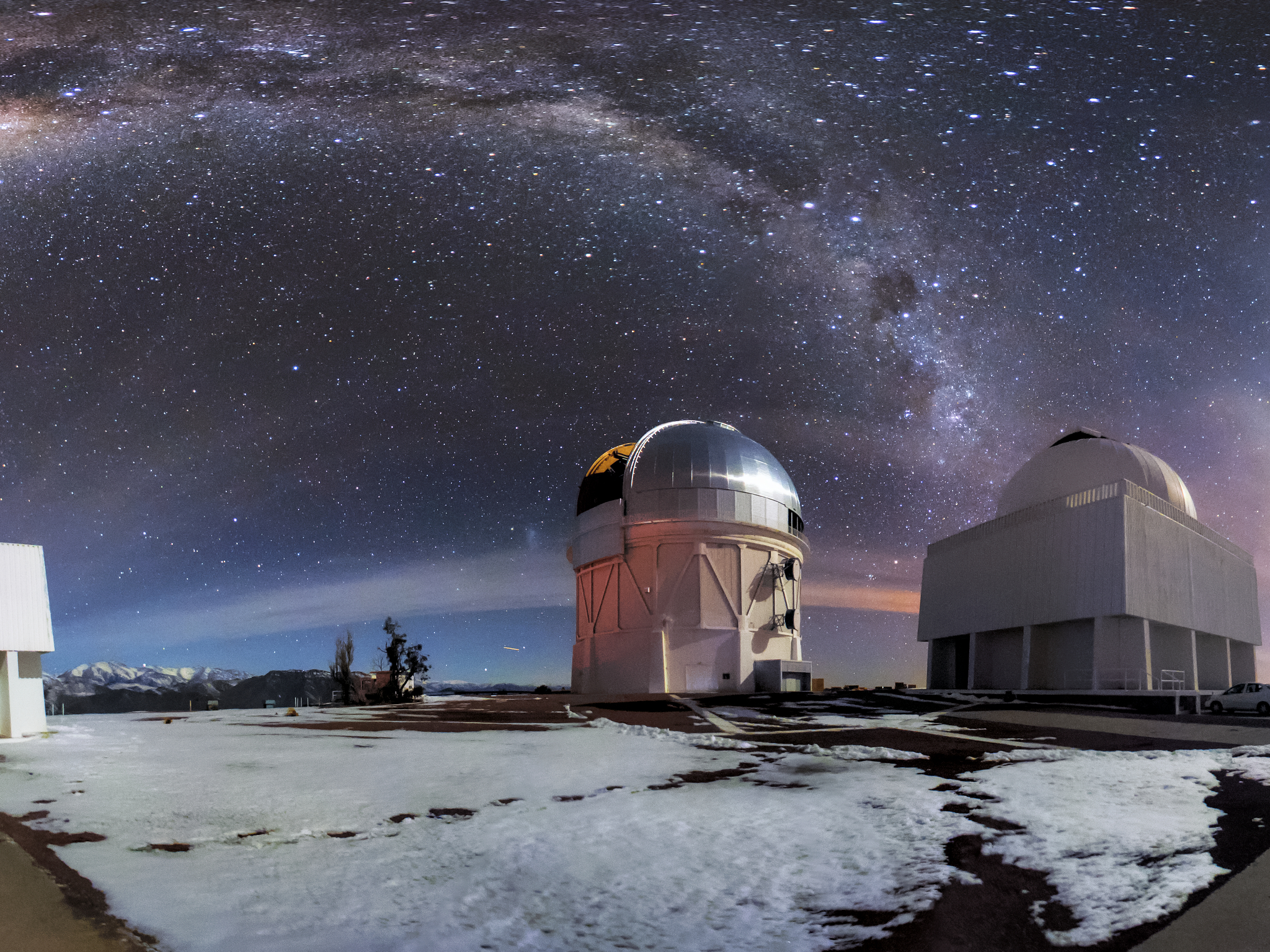The image captures an outdoor scene from a mountain peak where a space observatory, featuring a couple of buildings and telescopes, is situated. The main observatory is a round-shaped building with a silver dome, partially retracted to reveal the telescope, while another traditional rectangular building with a white dome sits to its right. The ground in the foreground has a light dusting of snow, and a pathway leads up to these structures. In the far-left background, snow-capped mountains and some trees are visible. Above the observatory, the night sky is ablaze with the starry expanse of the Milky Way, with millions of stars dotting the scene. The sky's lower portion shows a medium blue hue, gradually darkening to a deep navy, almost black, at the top. The photograph seems to be a time-lapse, as some stars exhibit a slight movement trail, reflecting the passage of time.